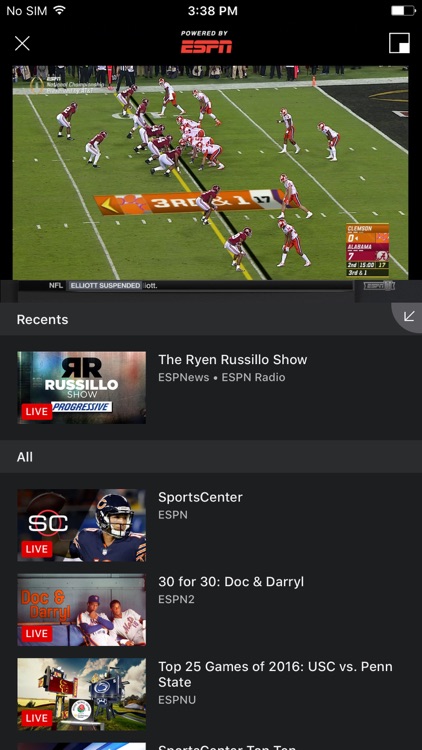This tall, vertically-oriented image, likely captured from an iPhone or Android device, is a screenshot featuring an ESPN video stream interface. At the very top, the status bar displays "No SIM" on the left, Wi-Fi signal icon, the time "3:38 PM" in the center, and a half-full battery icon on the right. Just below, there's a gray "X" button on the left and the text "powered by" followed by the ESPN logo in red at the center. To the right is an icon resembling a black square with a white rim and a smaller white square at the bottom right.

Occupying the upper third of the screenshot is a live scene from an American football game. The middle-lower portion of this segment features an orange line with an arrow pointing to the left, labeled "3rd and 1". The number "17" appears within a white line near a yellow "V" pointing left. Team logos are situated in a rectangular frame on the lower right: "Alabama" in red with its distinctive "A" logo, and possibly "Clemson" in faint orange and white text.

The bottom third of the screenshot includes various interface elements:
- A black bar with "NFL" in white letters, followed by white text on a gray background stating "Elliott suspended."
- A black bar on the far left with white text that's difficult to read, beneath which "Recents" is inscribed in white on a gray bar, paired with a downward-pointing white arrow.
- Below "Recents" is another gray area showing a rectangular thumbnail, labeled "RR" in black and white with "Relicio Show" in white letters on a red background to the lower left with the word "Live". The Progressive Insurance logo appears in black on a white background below "Show".
- On the right, another text reads "The Ryan Rufilo Show" in white, with "ESPN News" and "ESPN Radio" placed underneath in smaller text.
- Another gray bar to the left states "All" in white letters. 

Continuing below this section:
- A black background rectangle showing "SC" in white letters, with a red box containing "Live" in white, and a football player in a blue uniform and helmet pictured.
- To the right, "Sports Center" is written in white text with "ESPN" below it. Underneath, a square image shows two African American baseball players in white uniforms; the one on the left wears a blue cap. An orange "and" symbol followed by "Daryl" and further illegible text suggest "Dock and Daryl." The red "Live" box and white "30 for 30" text confirm the content as "Dock and Daryl, ESPN2".

Finally:
- The bottom section shows a billboard scene under a blue sky, with red and blue billboards and unrecognizable symbols. A red "Live" box is present in the lower-left. The white text reads "Top 25 Games of 2016, USC vs. Penn State, ESPNU."
- At the very bottom, a partially visible image and text are cut off and unreadable.